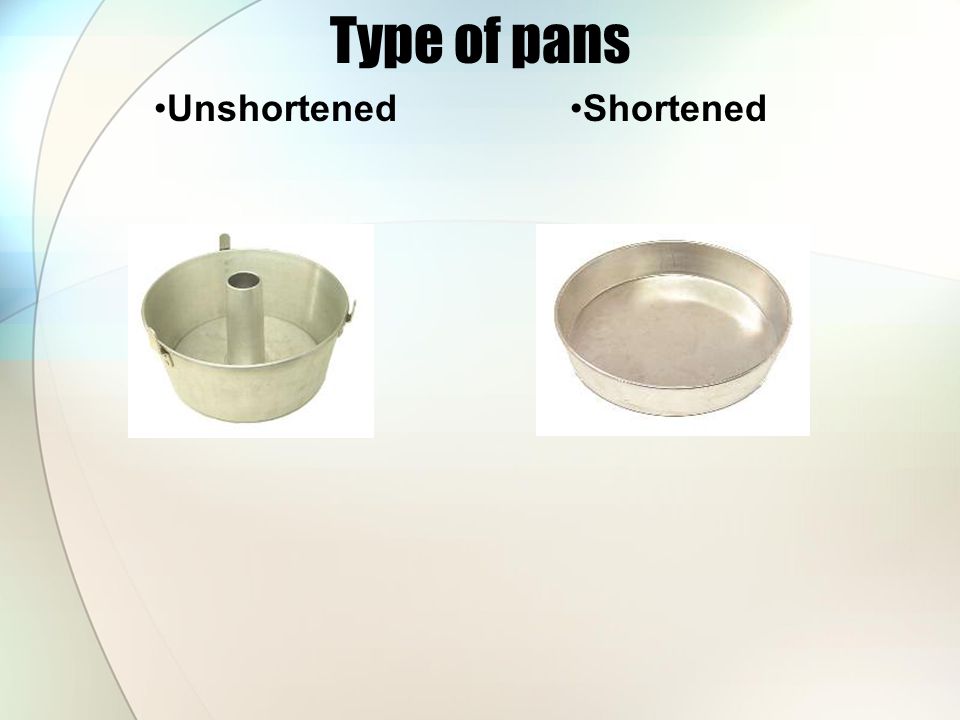This PowerPoint slide provides detailed information about different types of pans used for baking cakes. The slide features a background that is predominantly beige with gradual transitions to light blue and light green at the top, creating a subtle gradient effect. At the very top, the title "Type of Pans" is prominently displayed in capital and lowercase bubble letters. Below this title, the slide is divided into two sections:

On the left side, under the bullet point labeled "Unshortened," there is an image of a cylindrical silver metal pan, commonly known as an angel food cake pan or funnel pan. This pan features high sides and a central tube, designed to create a hole in the middle of the cake, ensuring even baking for unshortened cakes, which generally have a light, airy texture.

On the right side, under the bullet point labeled "Shortened," there is an image of a flat, circular silver metal pan with relatively low sides, typical of traditional cake pans. This pan is used for baking shortened cakes, which are known for their denser and moister texture. 

Both pans appear to have shiny edges, indicative of stainless steel or aluminum construction. Notably, the unshortened pan includes small clips, possibly for securing attachments or a lid, and both pans feature areas where lids could be placed. The overall layout ensures clarity and easy comparison between the two types of pans, against the gentle, complementary hues of the background.